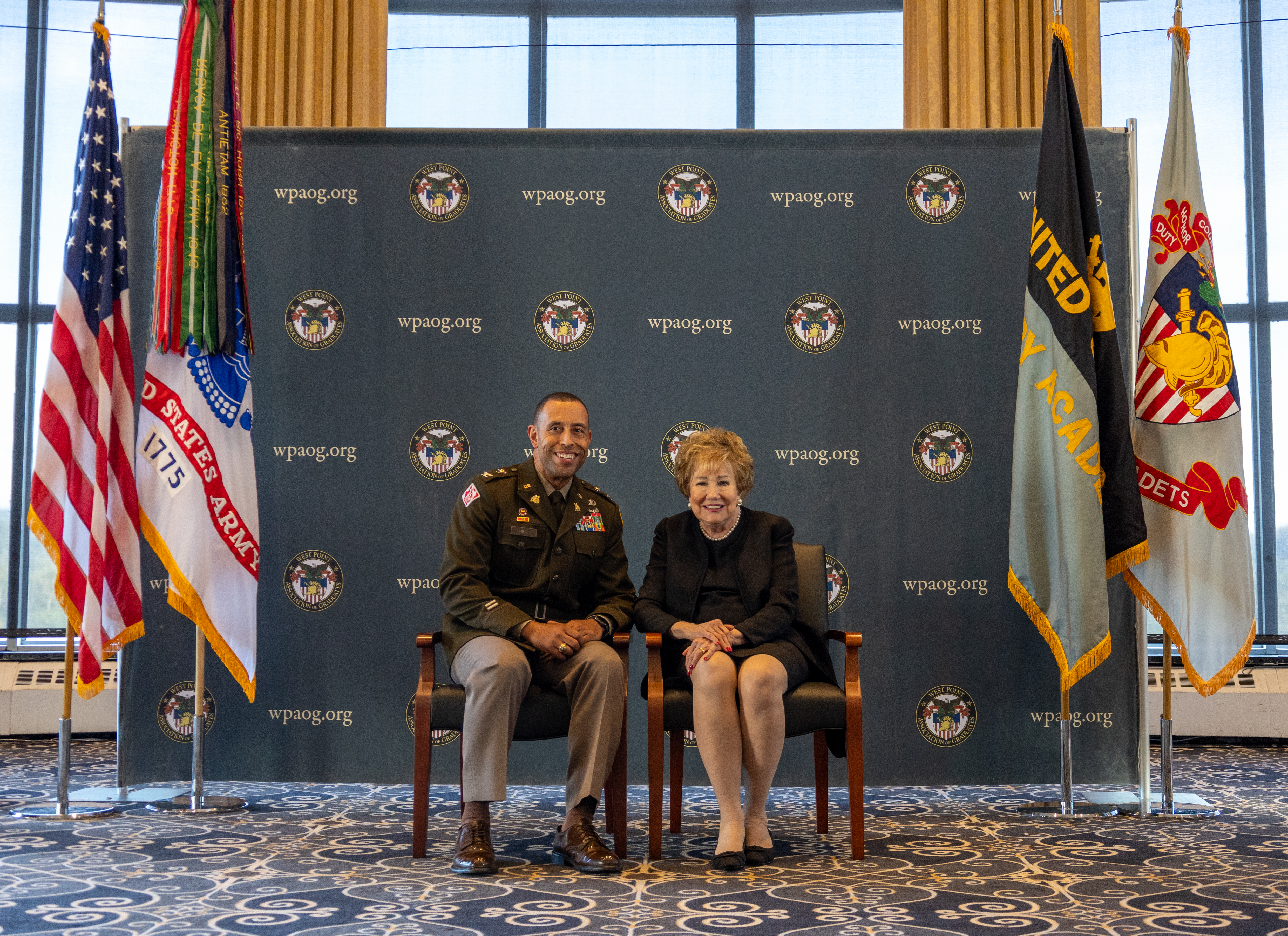In the image, we see a distinguished African-American man, possibly a former army sergeant, adorned in a military jacket decorated with multiple medals and patches. His attire includes gray pants and brown dress shoes. Seated beside him is a woman in her sixties, elegantly dressed in a black suit dress with pearl earrings and a pearl necklace, and black shoes. Both are sitting in stylish black chairs with reddish-brown armrests, leaning slightly towards each other.

The backdrop features a large board with the repeated logo and text "wpaog.org". Flanking this backdrop are multiple flags; on the left side, there is an American flag and another flag that reads "1775" with a shield resembling the American shield. On the right side, there is a gray and black flag and a white flag with green and red elements. The floor beneath them is covered with a blue and white floral-patterned carpet. Behind the backdrop, yellow curtains frame a wall of windows.